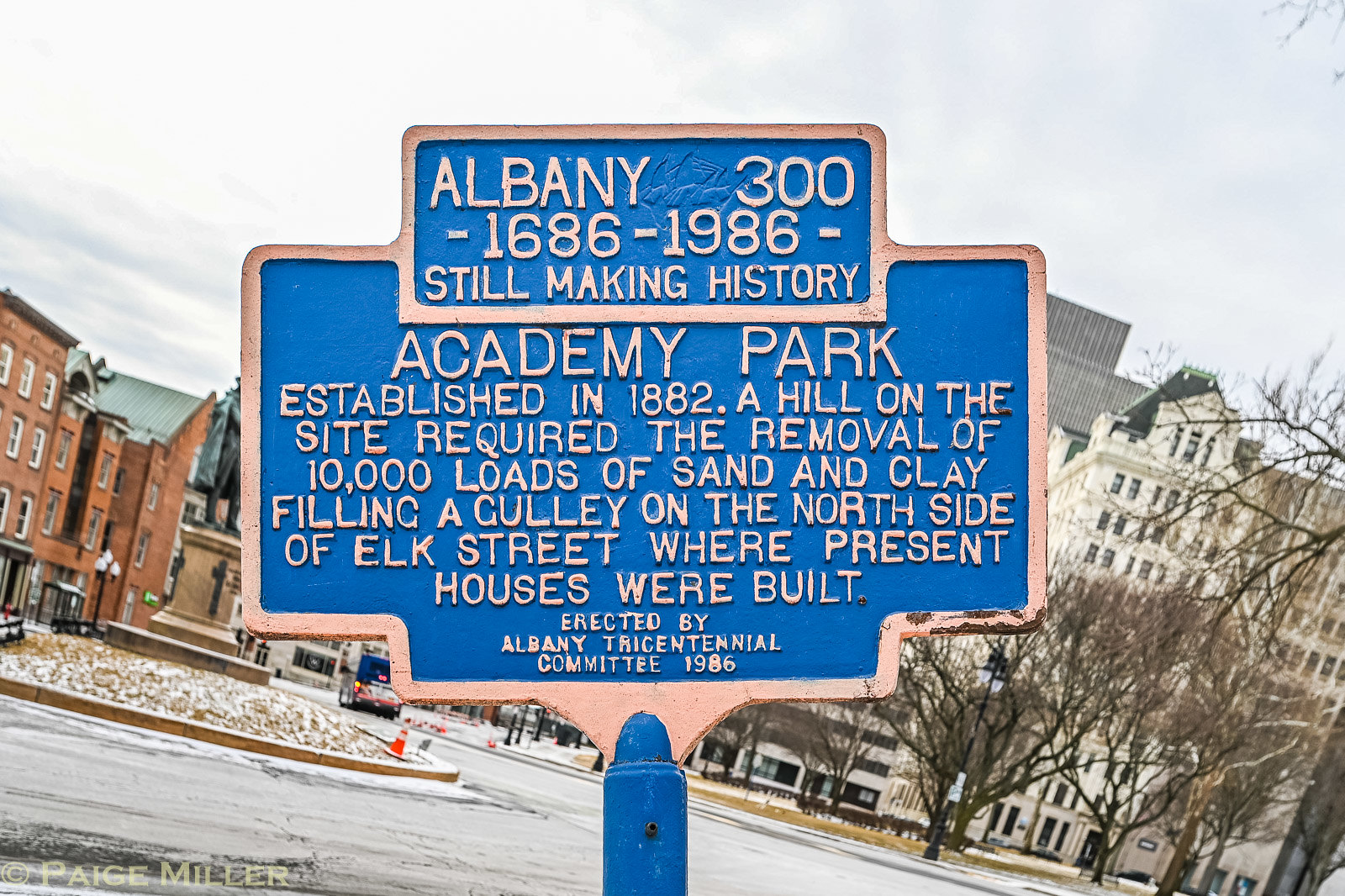In the foreground stands a weathered, blue metal plaque with a white border and white text, signifying the history of Albany. The plaque, mounted on a blue pole extending onto the street, reads:

"Albany 300, 1686 to 1986, still making history. Academy Park established in 1882. A hill on the site required the removal of 10,000 loads of sand and clay, filling a gully on the north side of Elk Street where present houses were built. Erected by Albany Tricentennial Committee, 1986."

Behind the plaque, a snowy cityscape unfolds. The background features buildings—both red brick structures to the left and newer, white-brick ones to the right—along with leafless trees and a roundabout containing a statue, partially obscured. The ground and streets are blanketed in snow, creating a clear winter scene. Except for the straight-standing plaque, the angled photograph makes the background appear somewhat tilted. The image, captured during the daytime under a cloudy sky, is credited to Paige Miller, noted at the bottom left of the plaque.